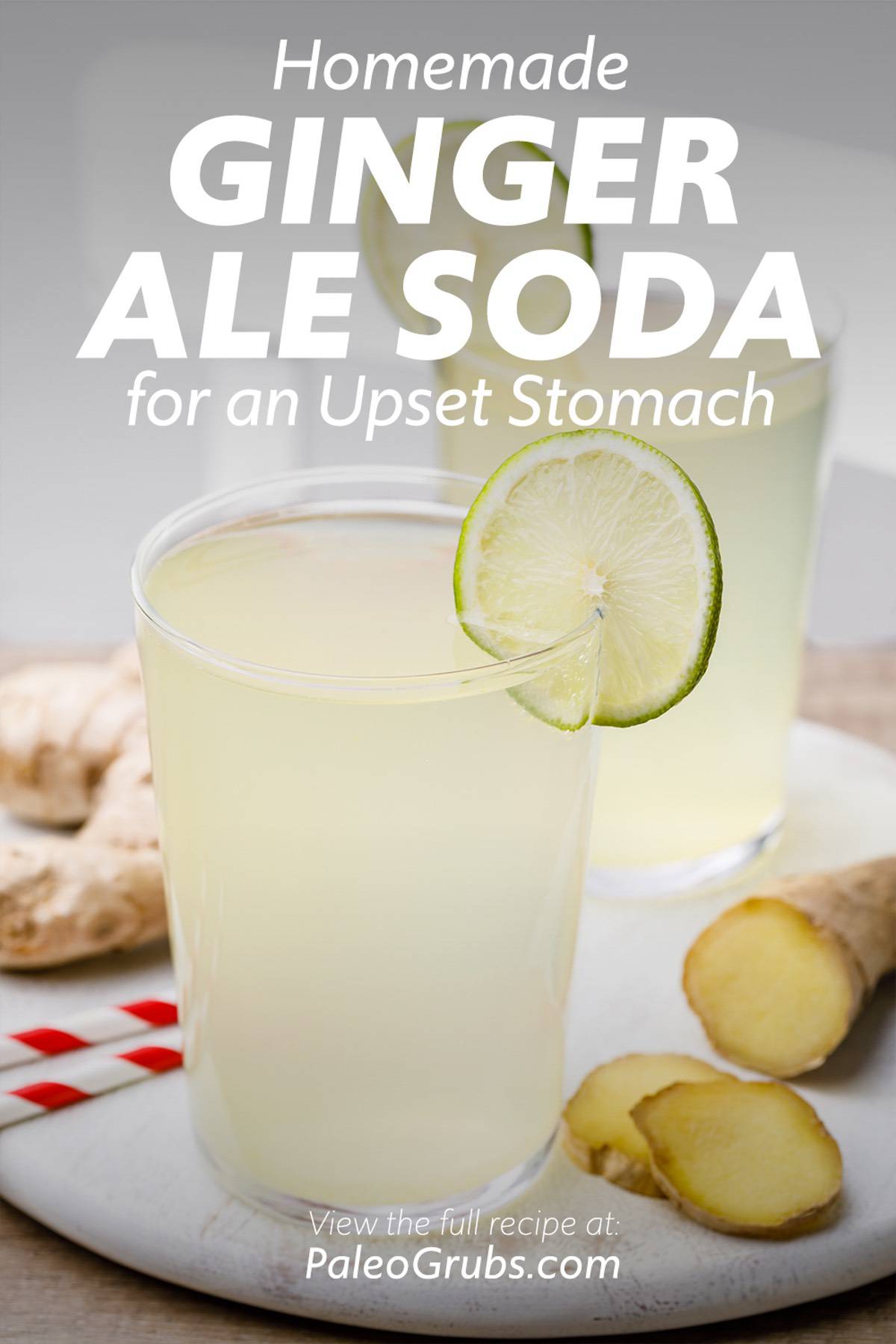The image is a detailed photograph showcasing two clear glasses of a pale, yellowish drink, identified as "Homemade Ginger Ale Soda for an upset stomach" in white text at the top. Both glasses feature lime wedges on their rims and are placed on a white plate. Flanking the glasses, the left side displays a whole ginger root, while the right side features ginger slices with two of these lying flat. Furthermore, two red and white striped straws are positioned on the left side of the glasses. The background is gray, and text at the bottom of the image reads, "View the full recipe at paleogrubs.com." The table on which the plate sits appears to be brown.